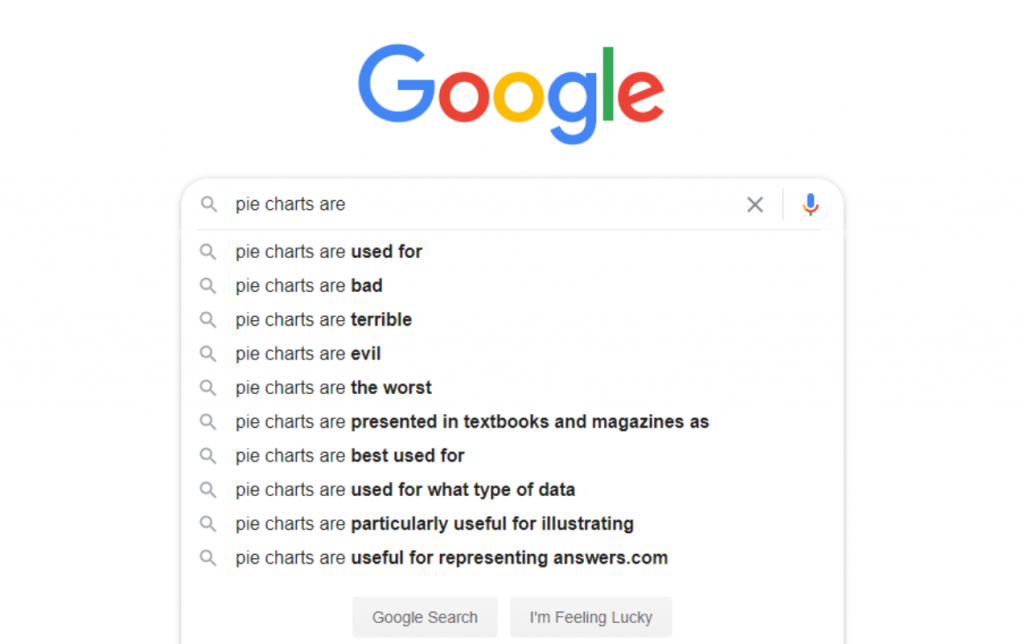In this rectangular image, we see a solid white background featuring a classic Google search page. Dominating the top portion, there's a large and colorful Google logo. Below the logo is a light gray search bar with the user's query "pie charts are" already typed in. Accompanying this search bar is a magnifying glass icon to the left. Underneath, a drop-down list of autocomplete suggestions appears, each prefixed with a magnifying glass icon. The suggestions read from top to bottom:

1. Pie charts are used for.
2. Pie charts are bad.
3. Pie charts are terrible.
4. Pie charts are evil.
5. Pie charts are the worst.
6. Pie charts are presented in textbooks and magazines as.
7. Pie charts are best used for.
8. Pie charts are used for what type of data.
9. Pie charts are particularly useful for illustrating.
10. Pie charts are useful for representing answers.com.